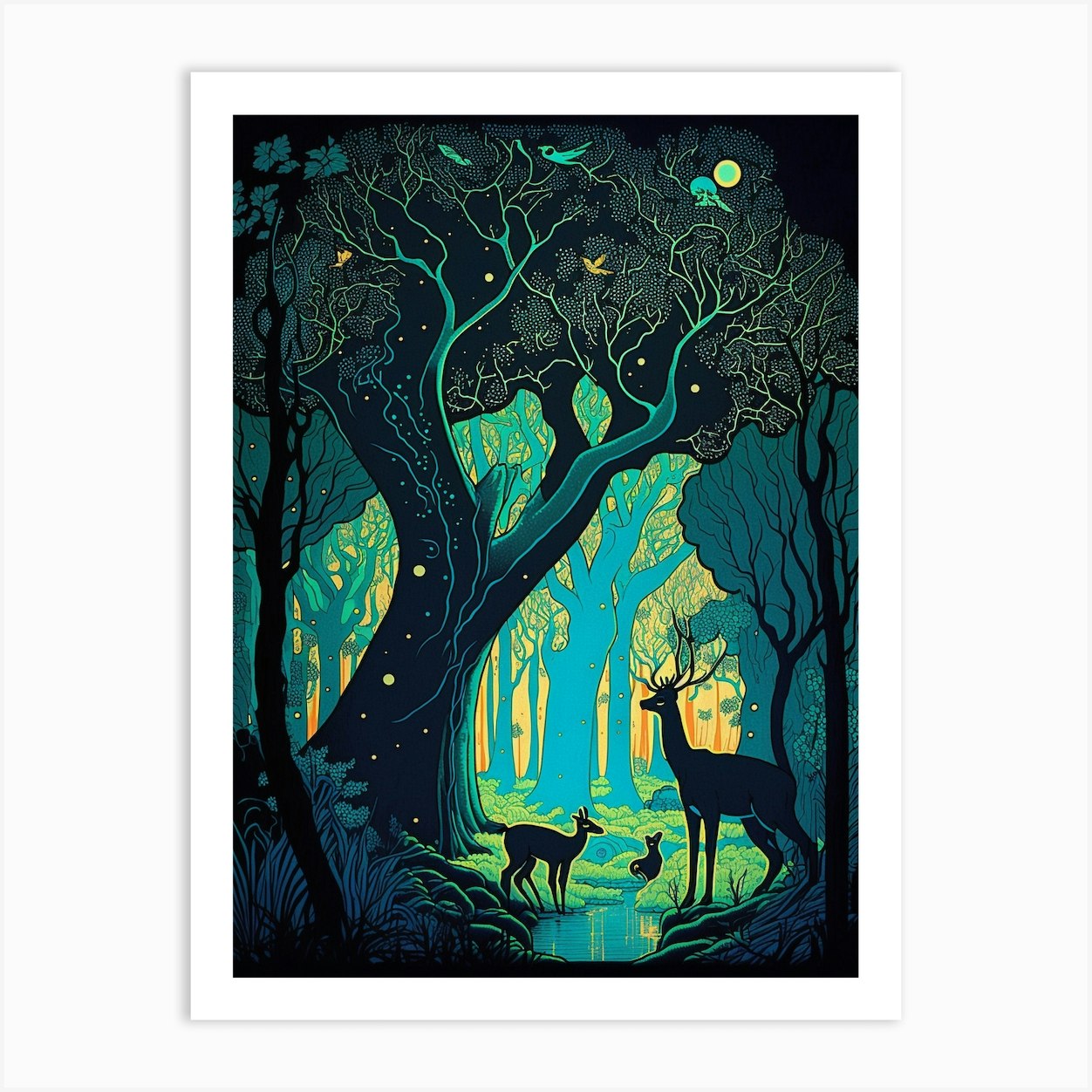This visually arresting painting depicts a mystical forest scene awash in a spectrum of dark and light hues. Dominating the scene is a large tree with a trunk painted in dark shades of navy and adorned with intertwining green foliage, standing to the left in the foreground. The artwork uses a mix of black, dark green, light green, and shadowy colors to evoke a nocturnal atmosphere. Contrasting the foreground, the trees in the distance have trunks in shades of light blue and are bathed in a gentle palette of light greens, suggesting an ethereal transition from night to day.

A white margin framing the image, mounted on an off-white wall, accentuates the contrasts within the painting. The expansive forest is inhabited by several deer silhouettes standing along the banks of a stream, which winds through the scene. In the foreground, a silhouetted buck with prominently displayed antlers stands to the right, while a smaller doe appears to be on the opposite bank of the stream. Additional details include a diminutive silhouette of a bird near the water's edge and a rabbit perched at the base of the tree.

Above, a celestial body, possibly the moon or sun, in shades of yellow and blue, adds a mysterious touch to the top-right corner, while the background gradually transitions into a soft glow of orange and yellow, evoking the break of dawn or twilight. The juxtaposition of dark and light elements within the forest gives the painting a timeless, almost surreal quality, inviting endless interpretations.